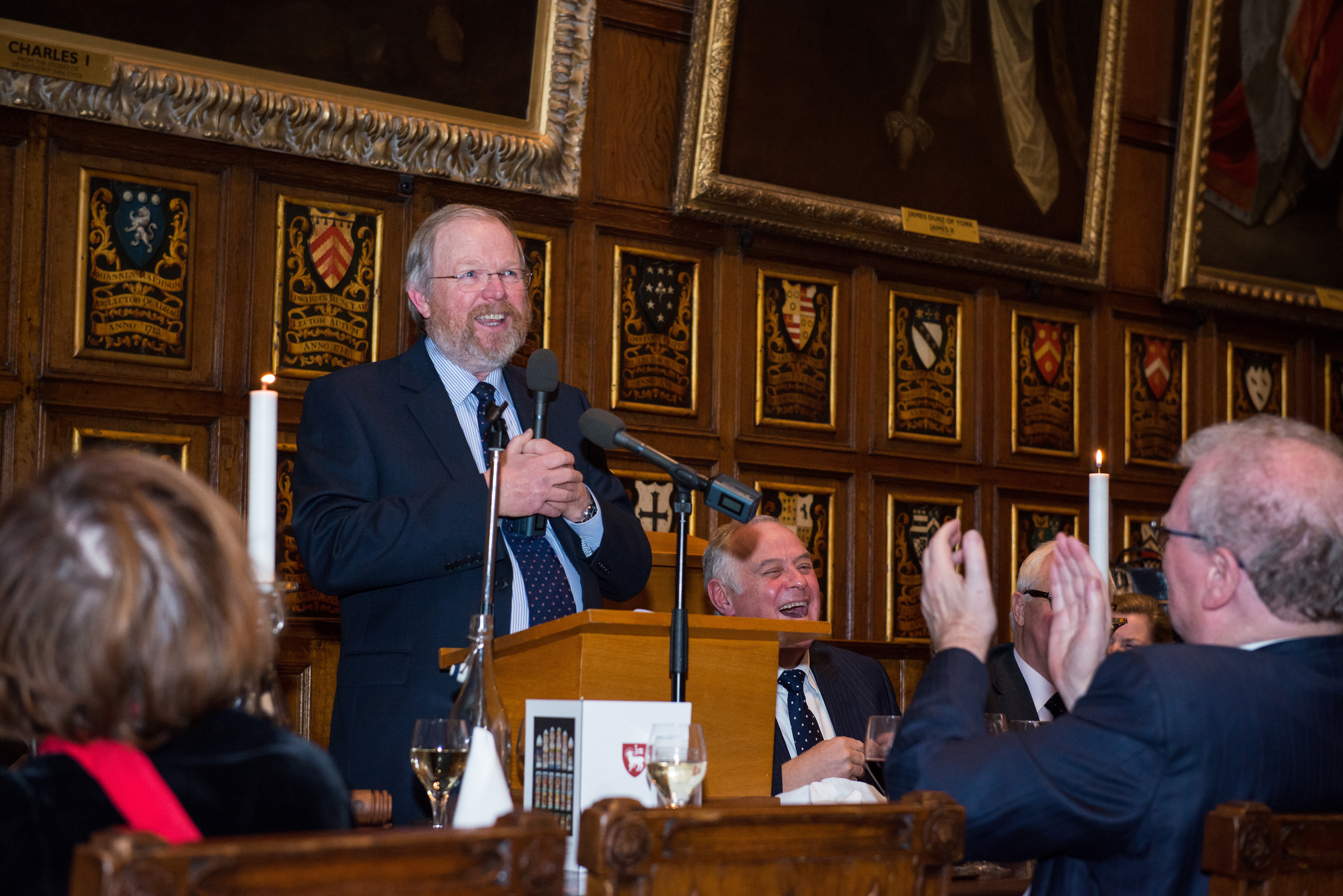The image captures an indoor setting where an older gentleman with gray hair, glasses, and a beard, dressed in a black suit jacket over a white or light blue collared shirt and a dark tie, is standing behind a brown podium. He holds a black microphone in his hands, smiling warmly as he appears to be making a speech. There is also a microphone on a black stand directly in front of the podium. To his left, another man, also in a suit and tie, with gray, balding hair, sits laughing. In the audience, people are clapping and appear to be enjoying the speech. Behind the speaker, the brown wall is adorned with numerous plaques in a row and large, valuable paintings in gold frames. The setting is well-lit, making the entire scene appear bright and clear. The men in the picture, who are likely in their late 70s to early 80s, exude a sense of celebration and camaraderie.